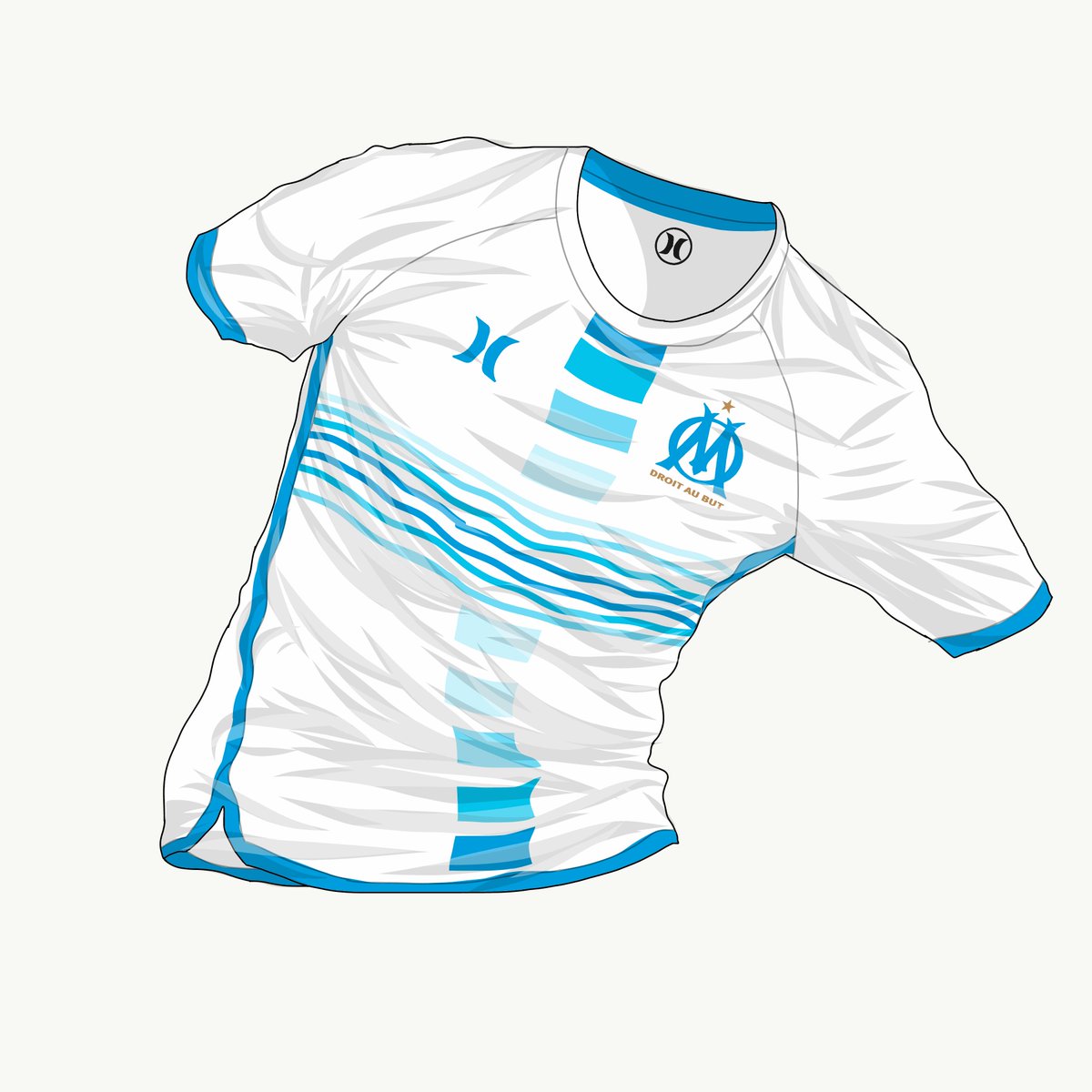The image showcases a digitally rendered soccer jersey set against a slightly off-white, eggshell-colored background. The object is precisely centered within the frame, resembling a product photograph one might find on an online clothing store. The jersey itself exhibits high-quality graphics, with no person wearing it, giving the illusion it has been laid out flat but with a dynamic twist, as if in mid-action.

The short-sleeve jersey prominently features a rounded neckline with a distinctive royal blue or teal blue band at the back of the neck and around the sleeve cuffs. The shirt's design is intricate, incorporating an array of colors—light gray, dark gray, white, various shades of blue and turquoise, and black. 

On the upper chest, two logos are present: on the left side, an 'H' formed by two inverted parentheses, and on the right side, a circular emblem containing an 'M' with an extending serif, accompanied by small, black text beneath it reading "DROIT ABOOT" and a gold star above. The front design includes vertical rectangles transitioning from darker to lighter shades of blue and back to darker as they approach the bottom. Additionally, there are seven thinner, horizontal stripes across the lower chest area, similarly transitioning in shades.

A singular blue stripe runs from the armpit down the sides to the bottom hem, which features slight openings where the front and back sides don't fully meet. Light gray areas are interspersed, simulating shadows and wrinkles, creating a lifelike depth and suggesting the jersey is in action.